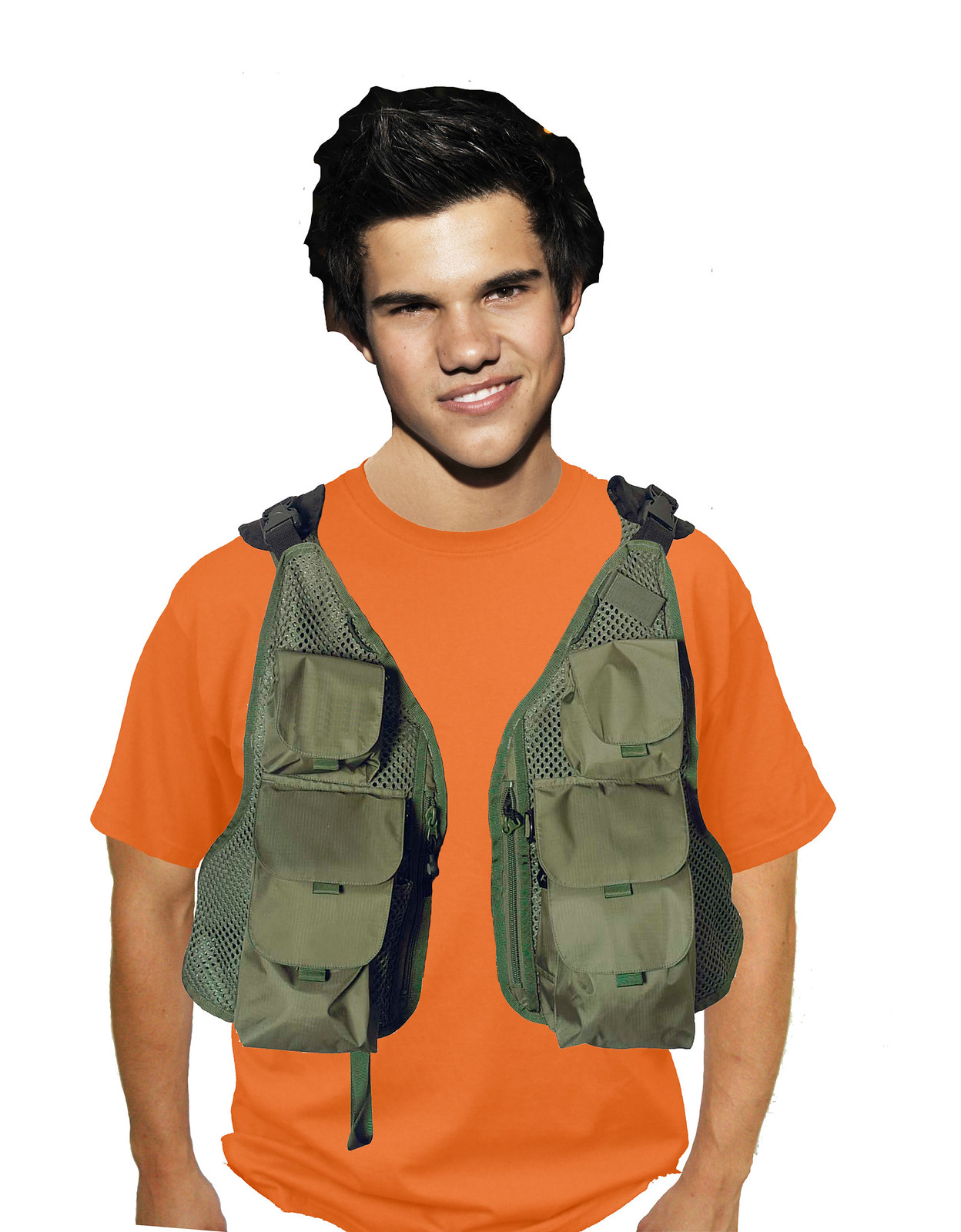This image features a photoshopped representation of a young Taylor Lautner against a plain white background. Taylor, known for his work as an actor, is depicted with a dark black, full head of hair, dark eyebrows, and dark eyes. He has a medium-light complexion, a wide nose, and a prominent chin framed by a bright white smile, with visible top teeth. He is dressed in an orange crewneck t-shirt and an olive-colored green mesh vest adorned with many pouches. The vest has three progressively larger pouches down the front of each side, secured with velcro, and features black buckles at the shoulders. While his arms hang down at his sides, from the elbows down, his hands and waist are cut off at the bottom of the image, highlighting the irregular edges typical of a Photoshop job.